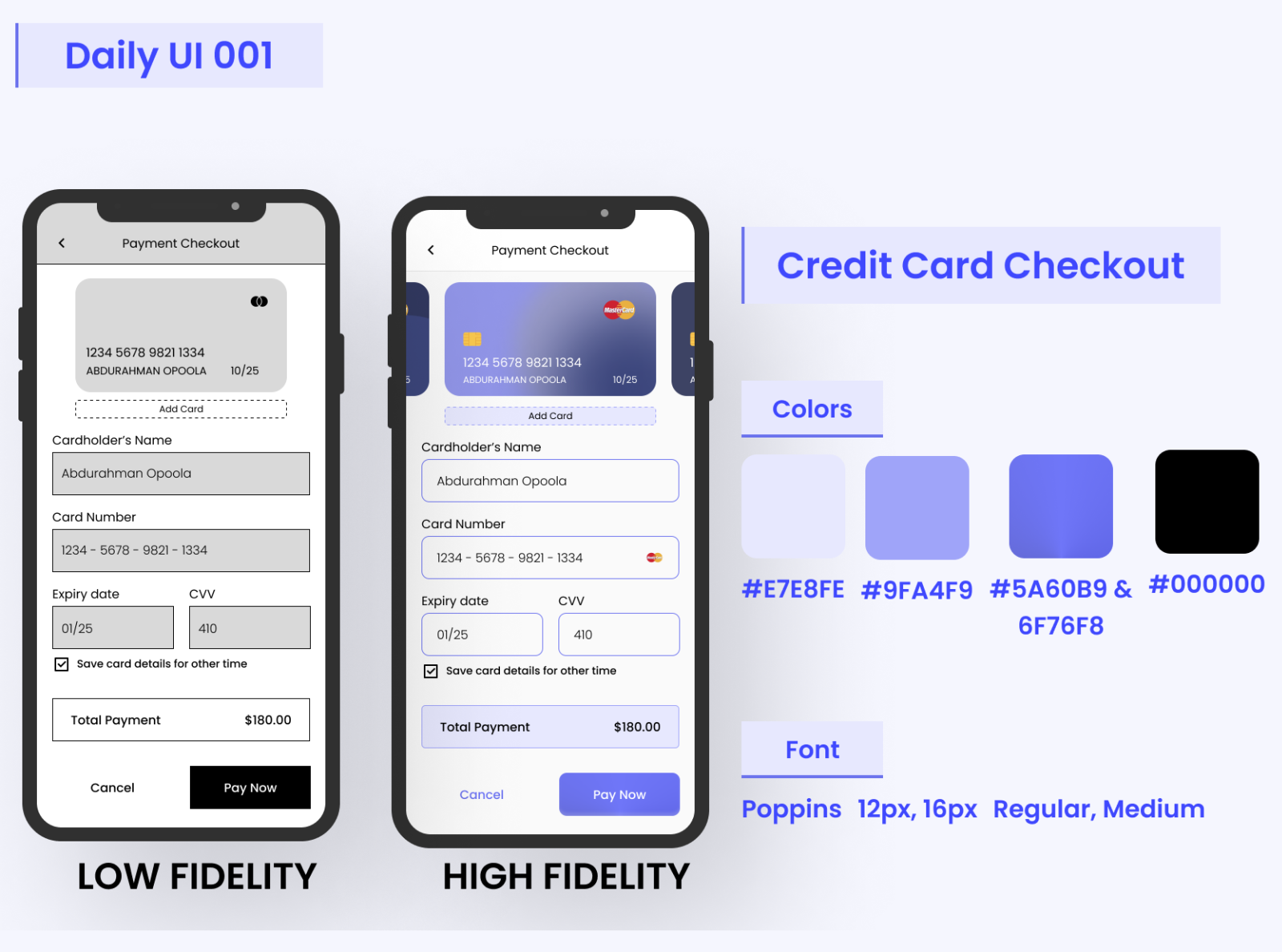In the top left corner of the image, the text reads "Daily UI 001." Below this header, there are two images of cell phone screens side by side.

On the left screen, which has a gray background, the header reads "Payment Checkout." Below this, various fields and options are displayed:
- A credit card icon in the upper right corner in black.
- Input fields for "Cardholder's Name," "Card Number," "Expiration Date," and "CVV."
- A checkbox labeled "Save card details for next time" which is checked.
- The total payment amount displayed as "$180."
- The text "LOW FIDELITY" is written in uppercase black text below.

On the right screen, the layout is similar but with differences in design:
- A blue credit card is shown, with the top-right corner displaying two circles—one red and one yellow—with the word "Mastercard" inside.
- The "Pay Now" button is blue.
- The text "HIGH FIDELITY" appears below the screen, in uppercase black text.

To the right of these images, additional design options are listed under the heading "CREDIT CARD CHECKOUT":
- "Colors" with choices of Light Blue, Medium Blue, Bold Blue, and Black.
- "Font" with choices listed as Poppins in sizes 12px and 16px, and styles Regular and Medium.

This detailed caption fully describes the visual and text elements present on the image.